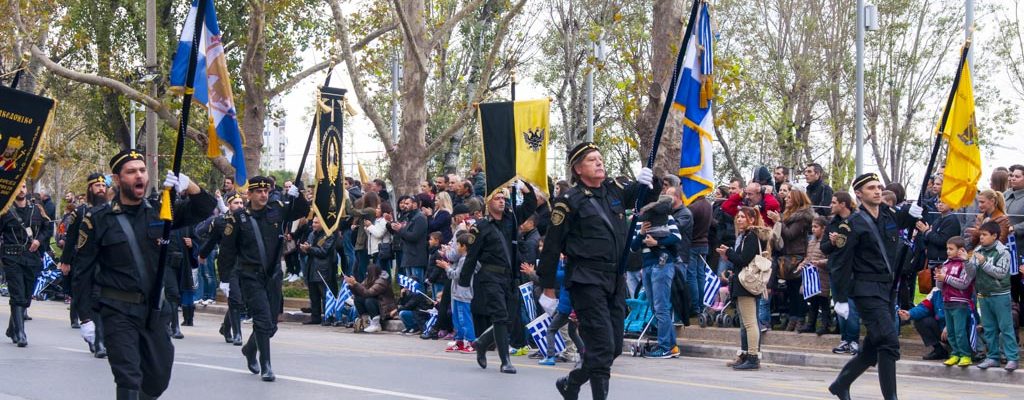This image showcases a disciplined group of soldiers, each adorned in black uniforms and black hats, adorned with distinctive patches on their arms and wearing white gloves, marching in a well-organized formation down a paved road. The soldiers are carrying a variety of flags, including prominent blue and white flags featuring white crosses and gold emblems, likely representing a specific country, possibly Finland, due to the resemblance to the Finnish flag. Additionally, there are black and yellow flags among them. One of the soldiers, positioned towards the left, appears to be shouting commands. The parade takes place beside a large crowd of enthusiastic spectators, who line the sides of the road, clapping and cheering for the marching soldiers. Some audience members are waving the country's flags, further enhancing the patriotic atmosphere. The backdrop features a row of trees, adding to the scenic setting of this possible military procession.